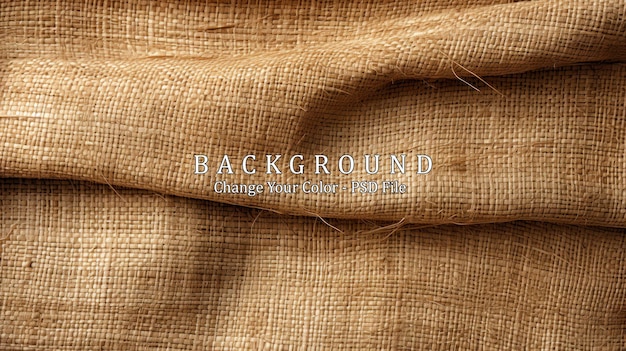This high-definition photograph captures an up-close view of a crumpled, tan-colored canvas material, which evokes the appearance of both woven flannel and twine. The rectangular image showcases the textured fabric with various-sized fibers interlaced, some of which are fraying and loose, reminiscent of rugged, weathered hay. The canvas is folded in multiple places, creating shadows beneath each crease. These creases and the evident wear give the material an old, almost deteriorating look. Centrally positioned in the photo, white text in all caps reads: "BACKGROUND, CHANGE YOUR COLOR, PSD FILE," standing out against the textured, rustic backdrop.